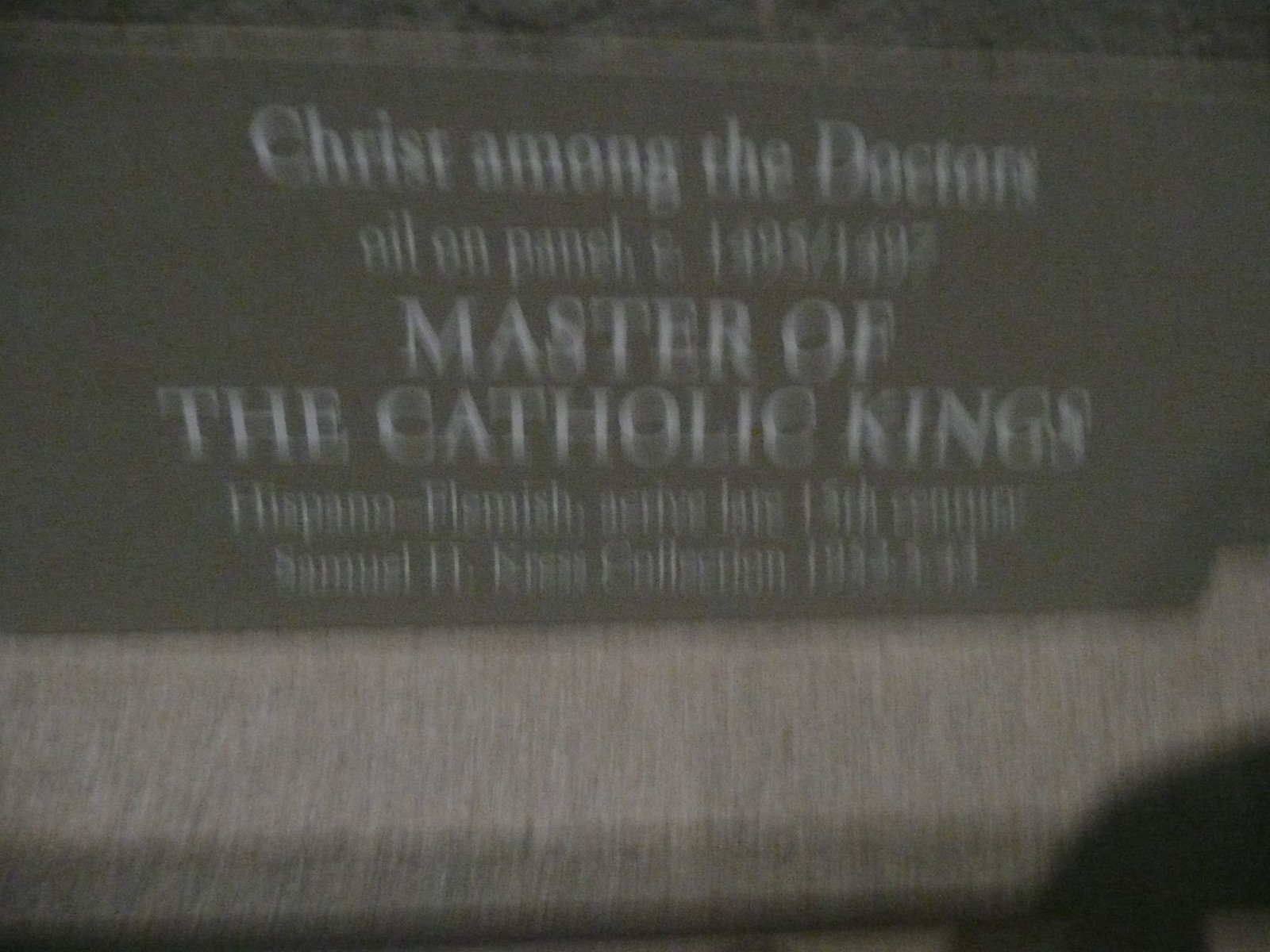This is a very blurry photo taken with a camera, depicting a gray, tombstone-like plaque at a museum. The plaque describes a painting entitled "Christ among the Doctors, Oil on Panel," attributed to the Master of the Catholic Kings, a Hispano-Flemish artist active in the late 15th century. The approximate dates given are circa 1495 to 1497. The text includes the Samuel H. Kress Collection, noted from the years 1953-54. The letters on the plaque are in white, making it stand out against the gray background.